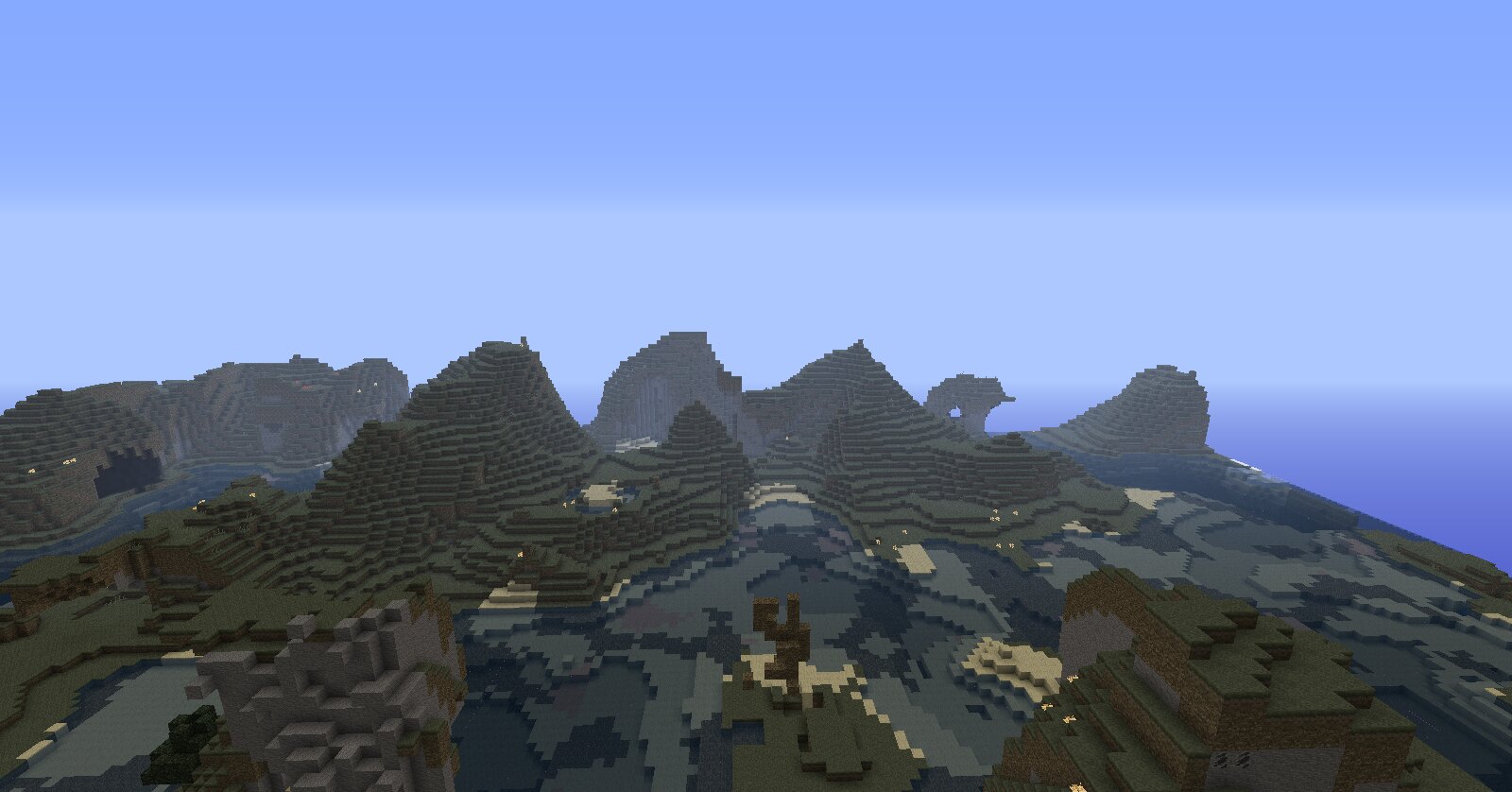The image is an aerial, pixelated view that vividly resembles a scene from a video game like Minecraft. It showcases an expansive range of cubular-shaped mountains set against a strikingly blue sky that fades from a darker shade at the top to a lighter hue in the center, and eventually transitions into a deep blue suggesting the presence of an ocean in the background. To the upper left, a river can be seen winding through a mountain pass, adding depth to the landscape. The surrounding areas are composed of escalated plateaus in varied colors including dark gray, light gray, tan, olive green, brown, and camouflage hues, which might imply forestry or different land textures. Though no buildings are clearly visible, the diverse coloration of the landscape hints at possible human habitation within this detailed, virtual terrain. Overall, the scene captures the intricate, blocky aesthetic typical of a digitally-rendered video game world.